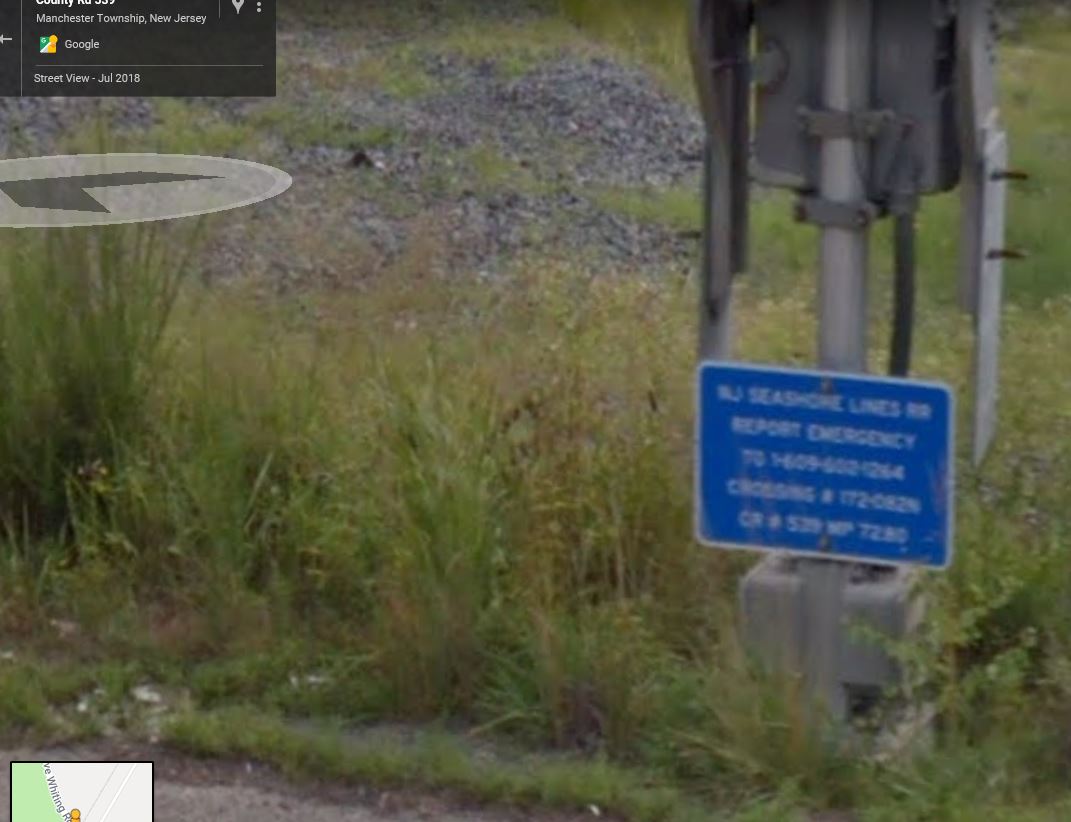The image appears to be a Street View snapshot from Google Maps, taken in July 2018 in Manchester Township, New Jersey. Dominating the scene is an electrical pole with a sign that reads "New Jersey Seashore Lines, RR, report emergency" followed by a phone number, though the number is too blurry to discern clearly. In the foreground, there's a grassy area leading to a gravel section in the background. The landscape inclines downward from the left side of the image to the right. Additionally, in the lower left-hand corner, there is a portion of the Google Maps interface, showing the top of the navigation icon commonly referred to as the "pegman." The upper left-hand corner includes on-screen text indicating the location and date: "Manchester Township, New Jersey, Google Maps," accompanied by the words "Street View, July 2018" and an arrow pointing to this section.